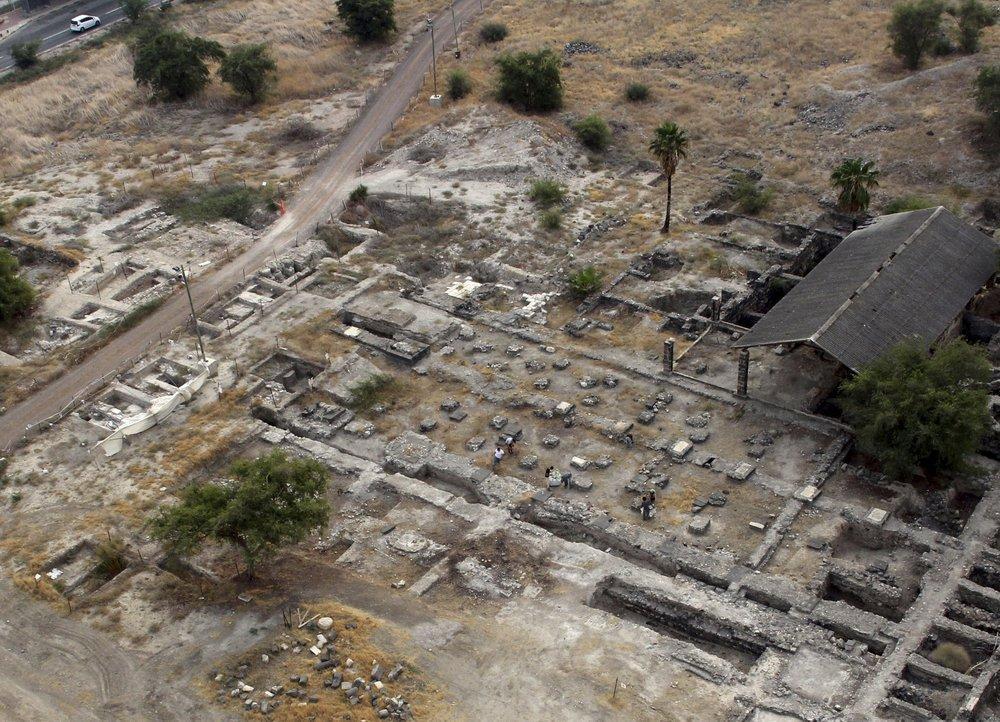This aerial image depicts an eerie, desolate scene, suggesting significant destruction or decay. The primary feature is a vast area covered in rubble and rocks, which was likely once a building or a cluster of buildings. The remnants of a single roof can be seen on the right-hand side, indicating that most structures have been obliterated by weather, construction, or perhaps an even more violent event. The landscape reveals a concrete base with geometric shapes and lines, which could suggest that this site might be an archaeological dig, where elements of the past are being methodically uncovered.

Scattered throughout the area, small figures of people can be seen, including a noticeable man in a white shirt, clustered around some of the stones, hinting at human activity amidst the destruction. The surrounding environment consists of both palm trees and scrubby vegetation, with colors dominated by browns, yellows, and sporadic greens from the trees. The top left corner features a white vehicle on a highway, adding to the contrast between the abandoned site and its surroundings. No specific signage or details are present to explain the history or purpose of the scene, amplifying its mysterious and somber tone.